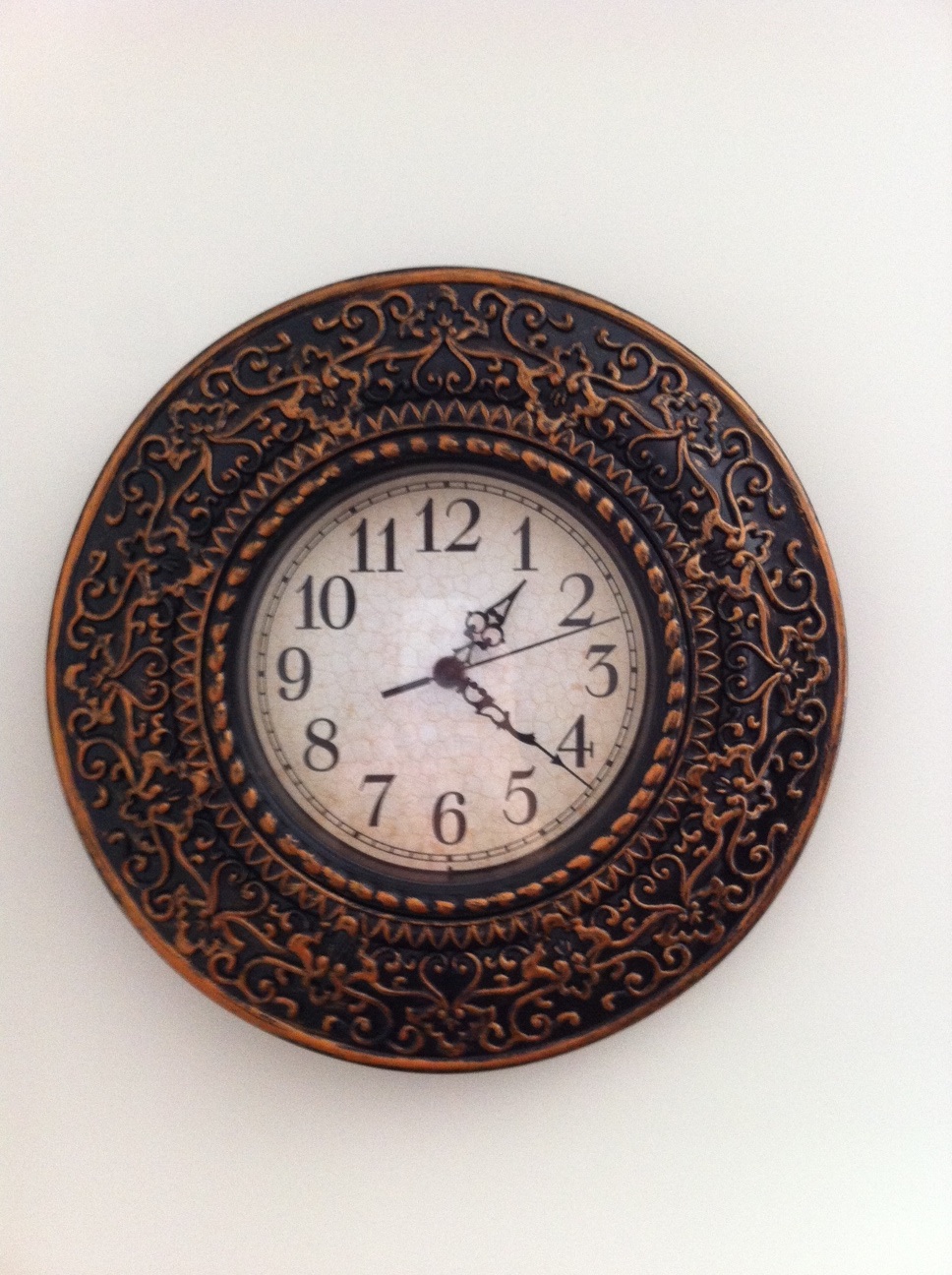This image showcases an antique wall clock centrally positioned in the frame. The clock features a white face with large black numerals, encircled by a black rim. Prominent black hands, including an hour, minute, and sweeping second hand, are highlighted with ornate scrollwork designs. The clock is set to approximately 1:22, with the second hand positioned between the two and three markers. The clock's border is a broad, hammered copper frame, aged to a dark patina, exuding a nostalgic character. This rich background is embellished with elegant brass scrollwork and a dimensional, layered design featuring an inner zigzag pattern and an innermost braided rope ring. All these intricate details contribute to the clock's vintage allure, making it both a functional timepiece and a decorative art piece.